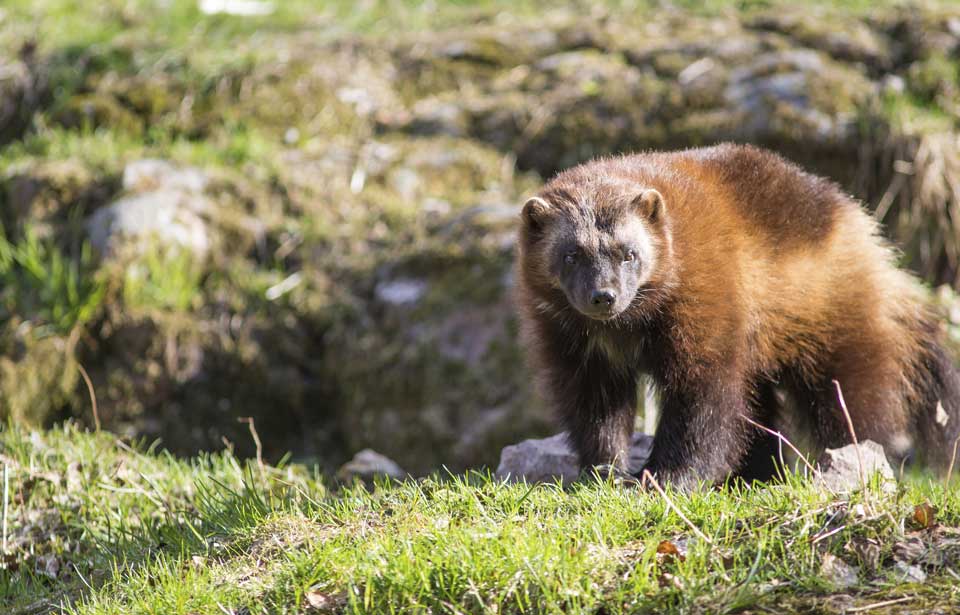This image depicts a four-legged mammal, likely a Tasmanian devil, in its natural habitat. The animal resembles a miniature bear with darker, fluffier fur. It stands on all fours on patchy grass and directly faces the camera with black eyes and a black nose. Its fur showcases a mixture of dark brown on its legs and rear, transitioning to lighter brown around its body, with faint white fur on its face. The setting is outdoors during daylight, featuring a nature backdrop of out-of-focus green foliage, white rocks covered in moss and grass, and scattered twigs. The animal is positioned possibly emerging from a pit or standing on a small hill, enclosed by rocks to its left and right.